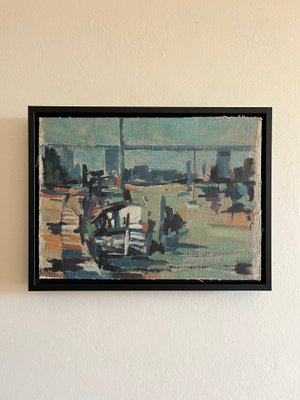This photograph captures a framed, impressionistic-style painting adorning a white wall, which appears slightly orange towards the top due to the lighting. The painting itself is rectangular, oriented horizontally, with a black frame. Dominated by abstract forms, it appears to depict a scene by a waterfront. On the left, vibrant orange hues frame what might be a small boat or houseboat next to a brick pier or walkway. Extending to the right, the scene transitions into green and blue tones, representing water and sky, respectively. The background showcases city buildings or a downtown skyline drawn in gray and blue, with tall, indistinct rectangular shapes indicative of skyscrapers. The brushstrokes are loose and undefined, blending elements together and creating a watercolor-like effect that blurs the boundaries between objects, light, and reflections.